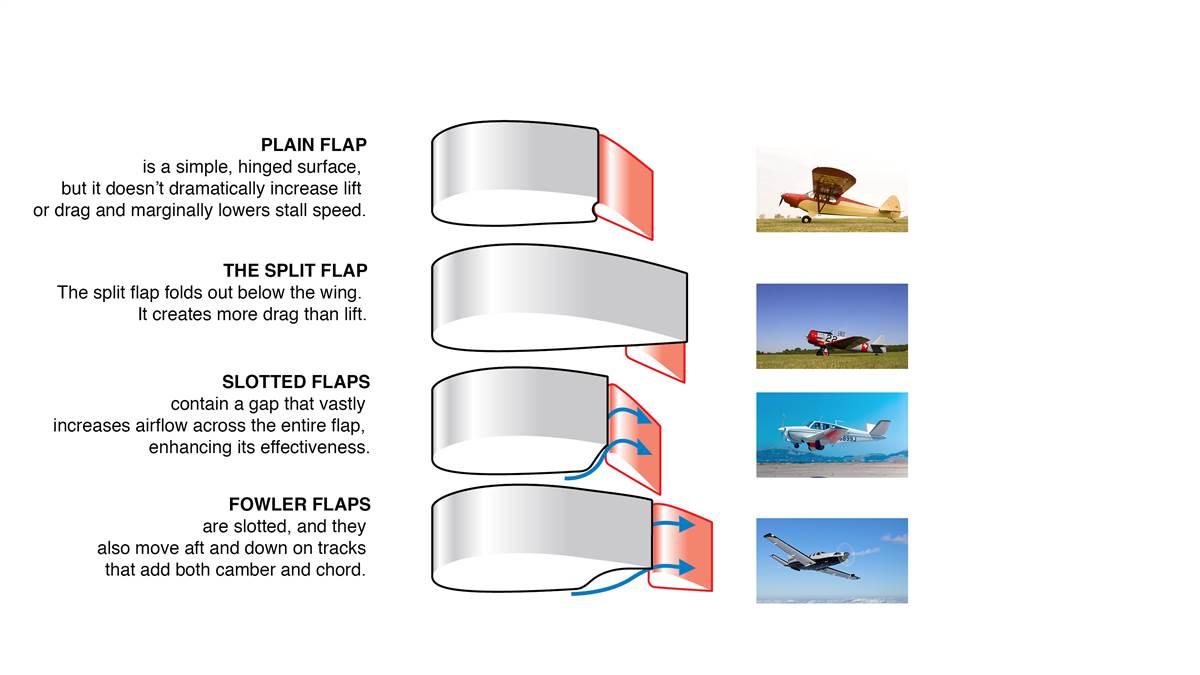The image is a detailed graphic, resembling a manual, explaining various types of airplane flaps on a white background. Along the left side, bold, capitalized names of flaps are listed, including Power Flap, Split Flap, Slotted Flap, and Fowler Flap, each accompanied by explanations in lowercase with punctuation. The center column features illustrations highlighting the distinct appearance of each flap. The far-right column displays photographs of different planes equipped with these flaps, linking specific flap types to corresponding aircraft.

Power Flap is described as a simple hinged surface, which does not significantly increase lift or drag, and marginally lowers stall speed. The Split Flap extends below the wing, creating additional drag and lift. Slotted Flaps contain a gap that increases airflow across the flap, significantly enhancing lift. Fowler Flaps are also slotted and move up and down tracks, increasing both camber and chord. The illustrations include markings like orange pieces and blue arrows to denote specific functions and movements.